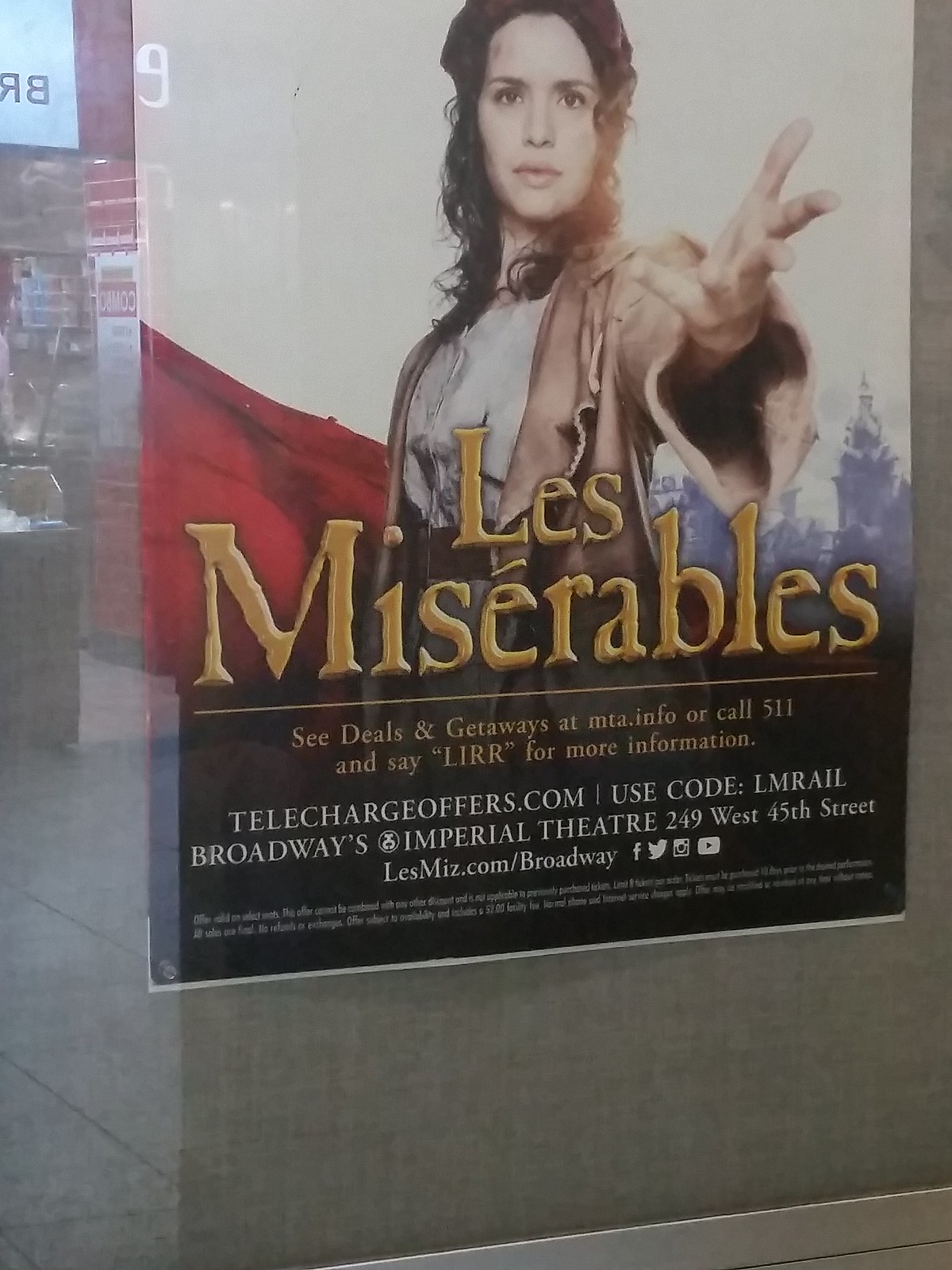Centered at the top of the poster, we see an image of a woman looking directly at us, her left hand outstretched with fingers spread. The background is a dark sky and, on the left side, approximately halfway down, there appears to be a red flag. The right side of the background showcases several buildings. Dominating the middle of the poster, in large font, is the title "LES MISÉRABLES."

A thin yellow line runs horizontally across the poster beneath the title. Below this line, in yellow letters, the text reads: "CD DEALS and GIVEAWAYS at mta.info or call 511 and say LIRR for more information." 

Further down, in all capital letters, it states: "telechargeoffer.com, use code LMRAIL, Broadway's Imperial Theater, 249 West 45th Street, lessmiss.com/broadway."